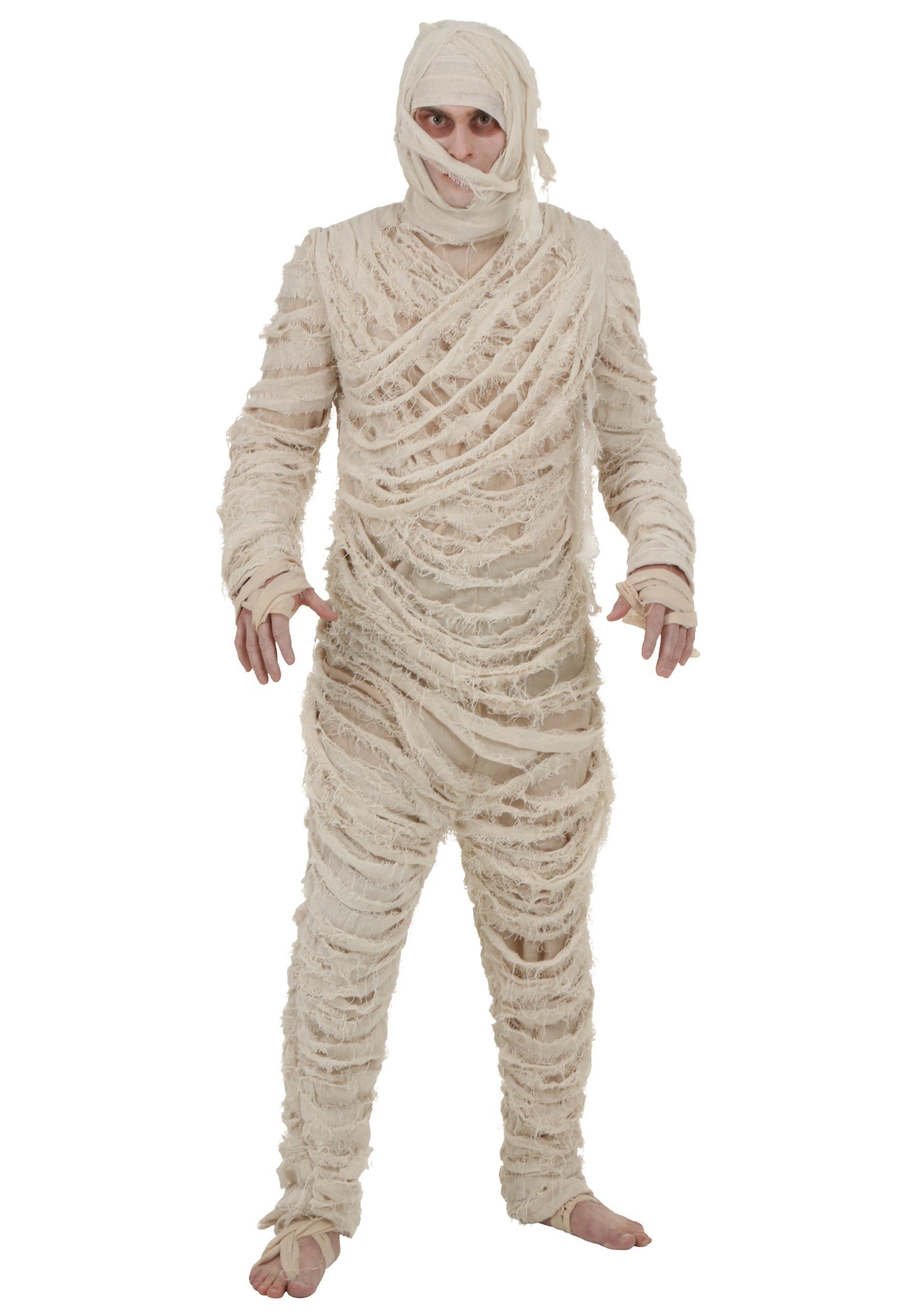The image portrays an eerie scene of a man resembling a mummy, situated against a stark white background that enhances the overall chilling effect. The mummy's body is enshrouded in loosely yet meticulously wrapped gauze and torn cloth, which look well weathered but not excessively tattered like in typical cartoon depictions. His uncovered skin, notably pale and dusted with white powder, peers through gaps around his nose, eyes, and a few fingers, adding to the haunting atmosphere. Notably, a strip of gauze stretches diagonally across his face, from under one eye and across his mouth to the middle of his opposite cheek. His arms are slightly tensed and positioned marginally away from his sides, and he appears to be taking a step forward with his right leg. The wrapping extends from the top of his head down to his feet, leaving portions of his fingers and toes uncovered. His feet, partially wrapped to the arch with a piece of cloth between his big toe and second toe, enhance the spectral authenticity, making it look as though he is stepping off the page toward the viewer.